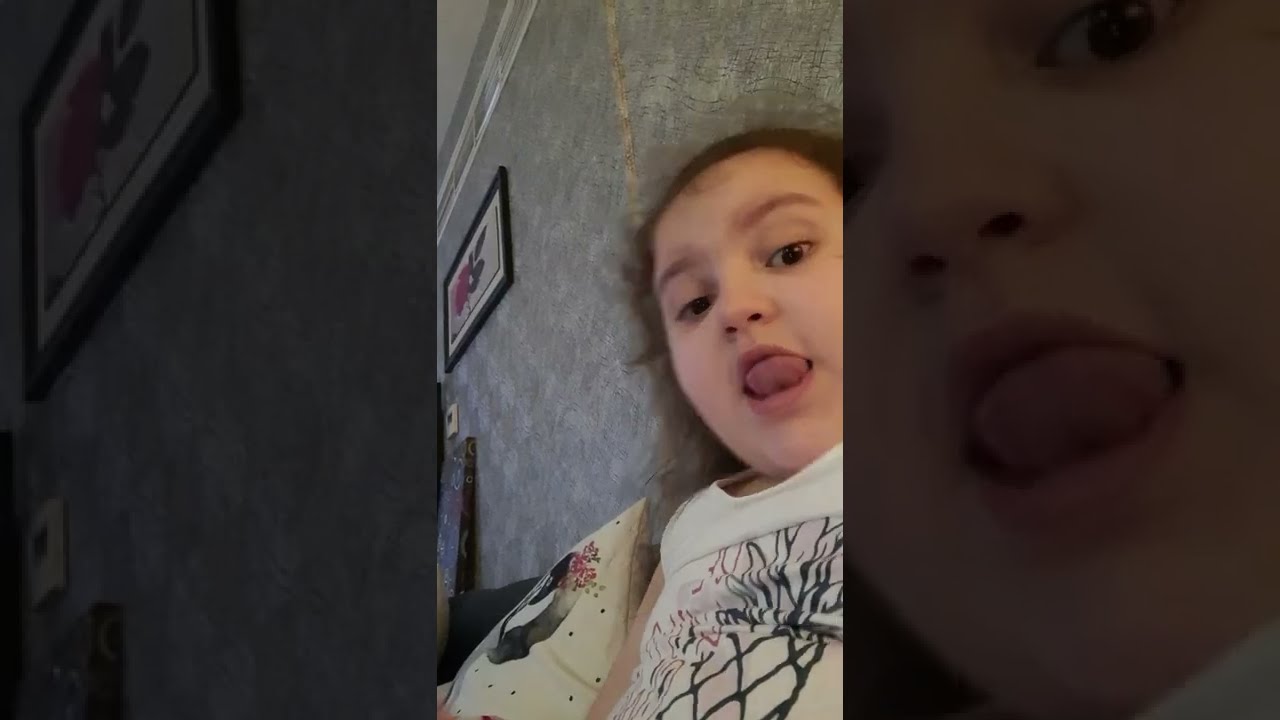This detailed photograph captures a young girl with dark brown, slightly frizzy hair, sticking her reddish tongue out towards the viewer. She wears a white tank top adorned with a black crisscross pattern, which might resemble branches. She is situated on a bed or couch, positioned against a textured gray wall. To her left lies a white pillow dotted with black spots, featuring a black and white bird-like figure, possibly a goose or a penguin, with a bouquet of pinkish-red and purple flowers. Above her, the ceiling appears white with a black-framed picture, and next to it, a white rectangular thermostat or device can be seen. The photograph has a tall, slim orientation, typically iPhone-like, with dark, grayed-out borders framing the image, zooming in on her expressive face and playful gesture. This intimate scene likely takes place in a bedroom, possibly her parents', capturing a moment of youthful spontaneity indoors.